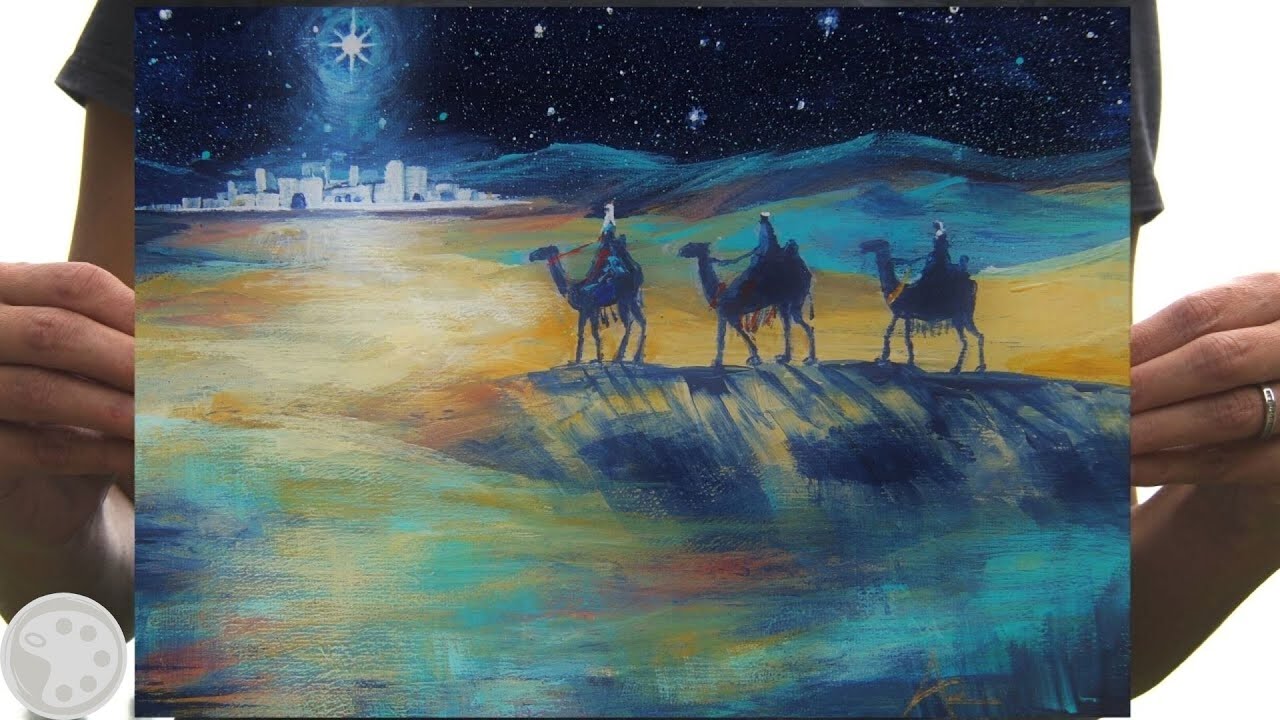The image is a color photograph showing a Caucasian woman, identifiable by her silver ring on the ring finger of her left hand and her short-sleeved gray top, holding up a painting against a white background. The painting, likely a reproduction, is a rectangular piece depicting a nighttime desert scene with broad strokes of greens, yellows, and blues. It features the three wise men on camels in a line atop a sand dune, their shadows stretching down the dune. The vast desert is illuminated by the large Star of Bethlehem, which baths a small city of white buildings below in a celestial glow. The sky is dotted with numerous stars with other dunes visible in the distance. This religious, Christmassy scene captures the moment the three wise men travel towards Bethlehem to visit the newborn Jesus, characterized by an abstract yet charming artistic style.